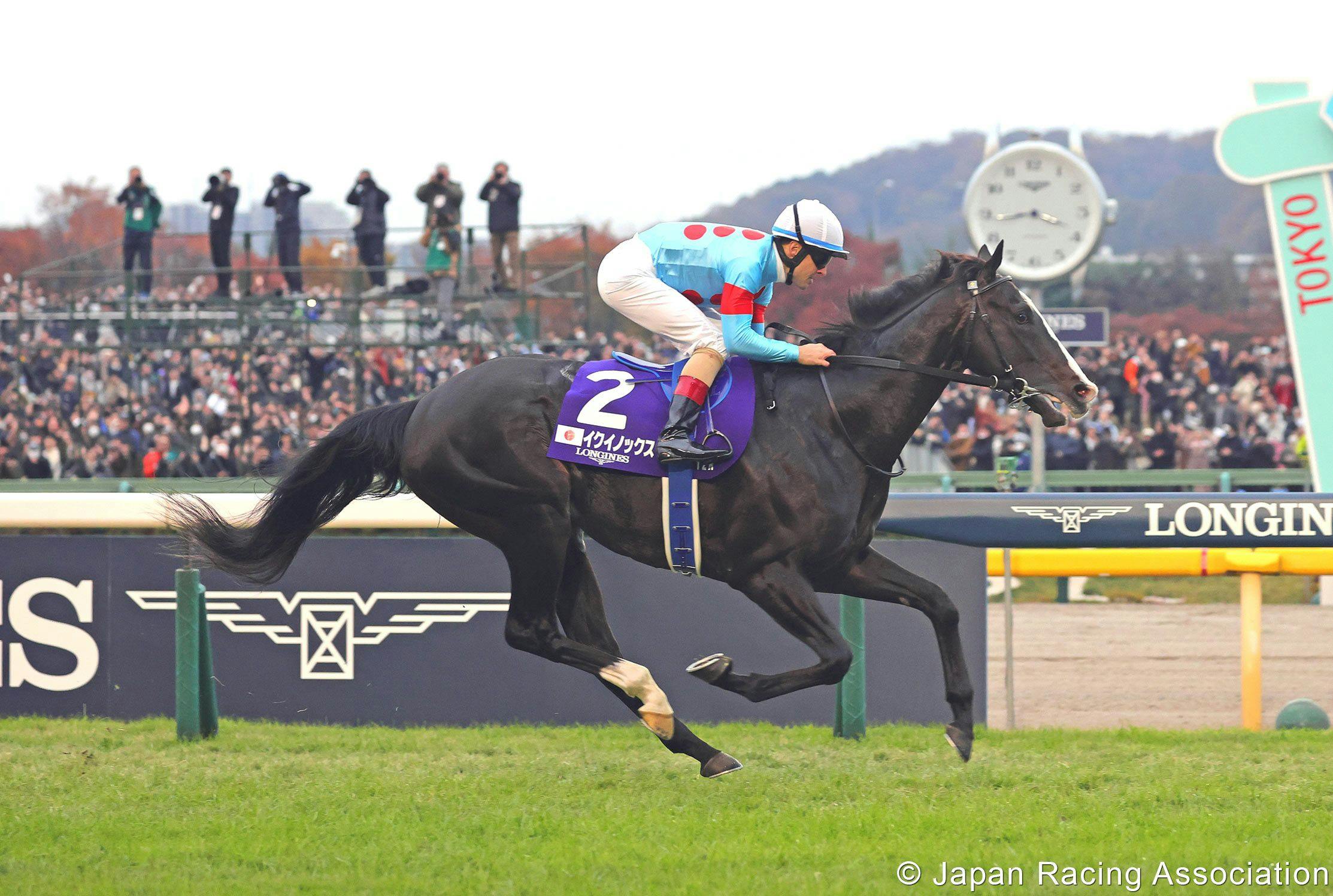The photograph captures the thrilling moment of a high-speed horse racing event, showcasing a dark brown horse with a distinctive white stripe running down its nose and a single white hoof. The horse, at full gallop on a lush, green grass track, seems to be almost airborne in its stride. A jockey, clad in a striking turquoise blue silk shirt adorned with three red dots down the back and a red armband, along with white pants, red socks, and black equestrian shoes, races with focused determination. The jockey's ensemble is completed by a white helmet trimmed in turquoise and black glasses. His saddle, marked with the number 2 and Japanese characters, prominently features the Longines logo. In the vibrant background, spectators eagerly watch the race, while photographers on an elevated platform capture the action. A large white clock and a partially visible "Tokyo" sign in red, set against a blue background, along with the LOGING logo on the fence, provide context to the setting, underscoring the event's connection with the Japan Racing Association, signified by a copyright notice.